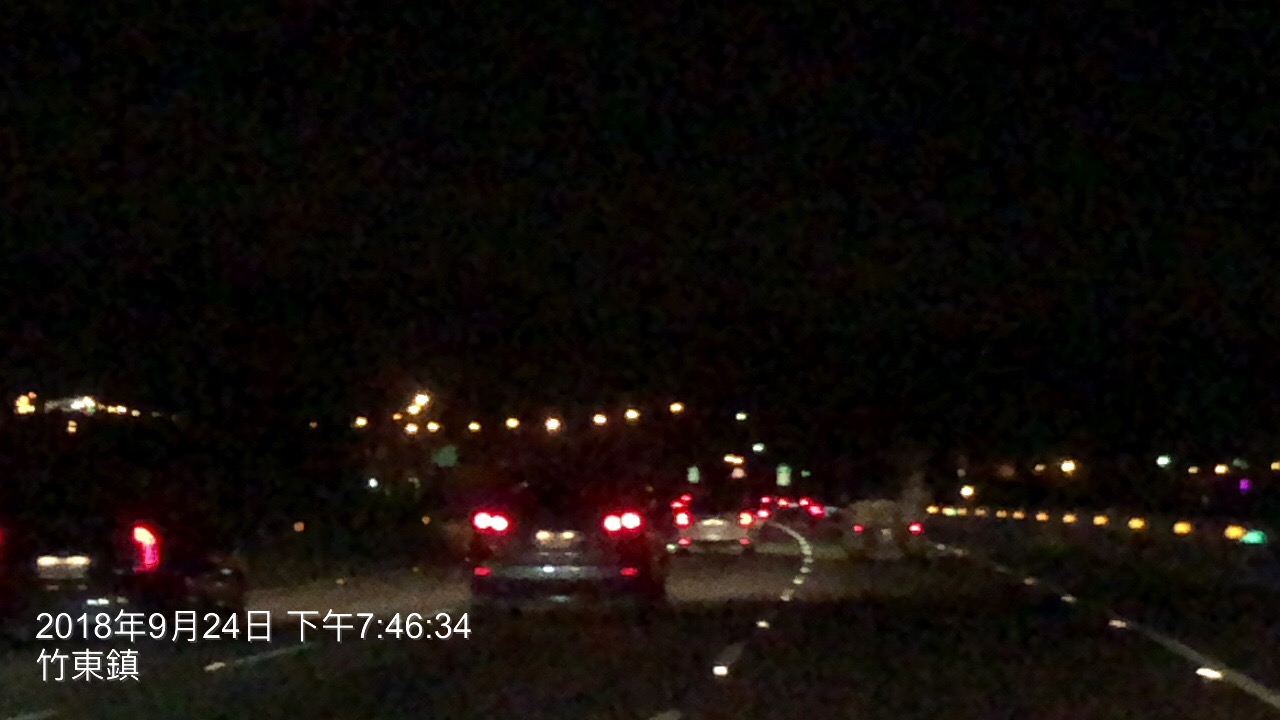A grainy dashcam photo captures a bustling late-night drive on a three-lane highway. The low-quality image, taken from a car traveling in the far right lane, suggests a busy road with six or seven visible vehicles as the highway gently curves to the left. Streetlights dot the horizon, illuminating the scene against the pitch-black sky, implying either a very late hour or a region where the sun sets early. In the bottom left corner, the timestamp "2018-09-24 7:46:34" is visible, accompanied by characters that appear to be in Cantonese, Mandarin, or Japanese, adding an element of mystery to the photo's origin.